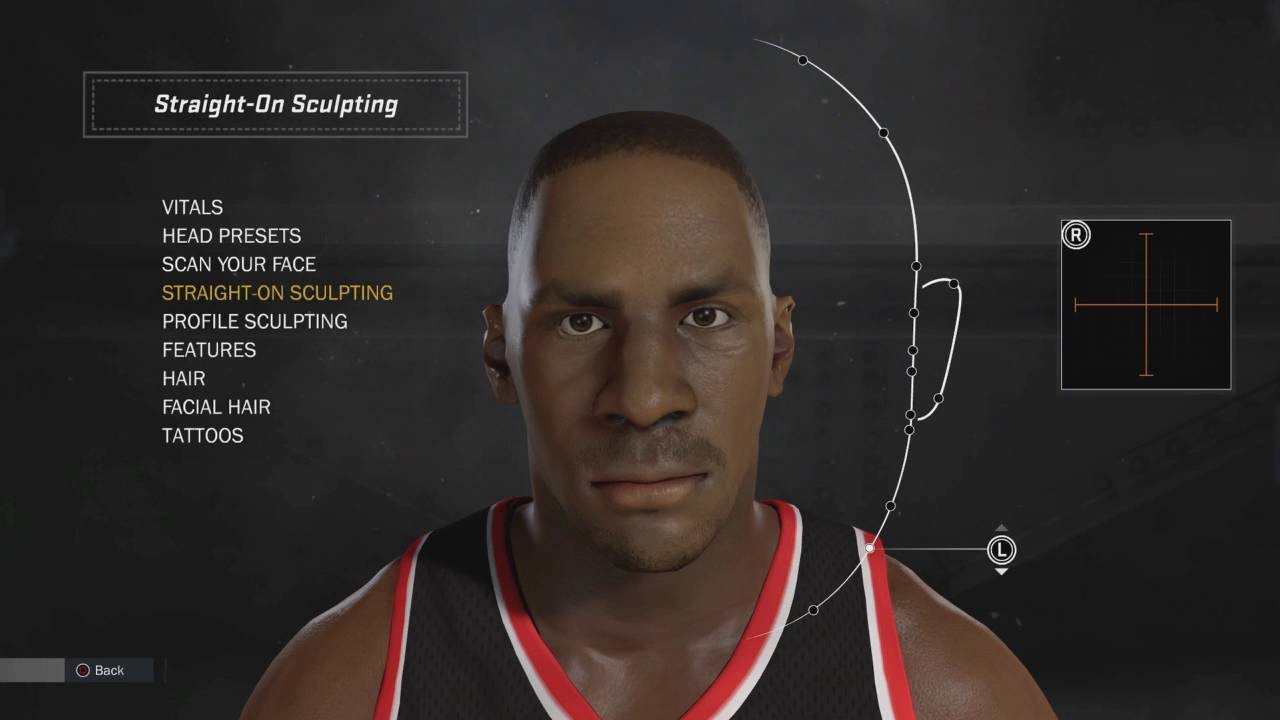A screenshot taken from a video game features a character creation screen. The background is a dark grayish black, and at the center is the head of an avatar resembling a Black man. The avatar has short black hair and a few days’ worth of stubble forming a thin mustache. The character has distinct facial features including black eyes, a prominent nose, and full lips. Due to the nature of video game graphics, the ears on either side of the avatar’s head look noticeably different.

The character is wearing a black jersey. Surrounding the head, there is an outline that appears to be in the process of being edited, giving it a slightly distorted appearance. In the upper left corner, a white rectangle contains the text "Straight on Sculpting". Below this are several menu options: "Vitals", "Head Presets", "Scan Your Face", "Straight on Sculpting" (highlighted in yellow), and lists for "Profile Sculpting", "Features", "Hair", "Facial Hair", and "Tattoos".

In the bottom left corner, there is a small gray rectangle next to a black one, inside which is a red circle containing the word "Back". On the right-hand side of the screen, there is an L-shaped icon inside a circle that indicates up and down movement. Near the upper right corner, there is a square with an "R" in a circle positioned in the upper left-hand corner of the square.